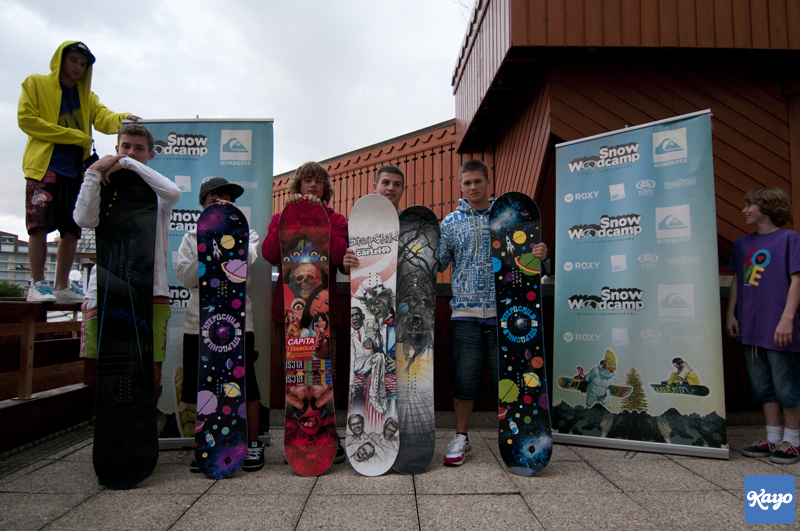The photograph showcases a group of seven adolescent boys, arranged in a row against an overcast sky. The boys are standing or positioned on grey tiles, indicating an outside setting with visible red roofing in the background. On the far left, one boy stands atop a fence or balcony railing, dressed in a yellow hoodie, black hat, and patterned shorts, with a blue shirt featuring green writing. Next to him, a boy in green shorts holds what appears to be a large snowboard or skateboard. The following boy, shorter than the rest, wears a white shirt, black shorts, and a hat, and holds a colorful board adorned with images of planets and vibrant colors like yellow, purple, and pink. Further to the right, another adolescent in a red shirt holds a red board decorated with faces and a skull. The next boy, whose clothing is not fully visible, is holding two boards, one predominantly white with black drawings of a crowned figure and suited person, and another board that's gray with intricate black lines. The succeeding boy is clad in a blue jacket and pants, holding a board featuring planets with blue writing in a circle. On the far right, another boy stands apart on the other side of a banner, smiling, dressed in a shirt with multicolored "Love" text and matching shorts, next to a blue square sign reading “Kale”.

All the boys appear happy, holding their distinctly designed boards. The scene is framed by two blue banners that read “Snow Wood Camp” multiple times, adorned with Quicksilver, Roxy logos, and illustrations of snowboarders. The detailed designs on the boards and the varied apparel of the boys add color and intrigue to the scene, highlighting elements of both winter and board sports culture.